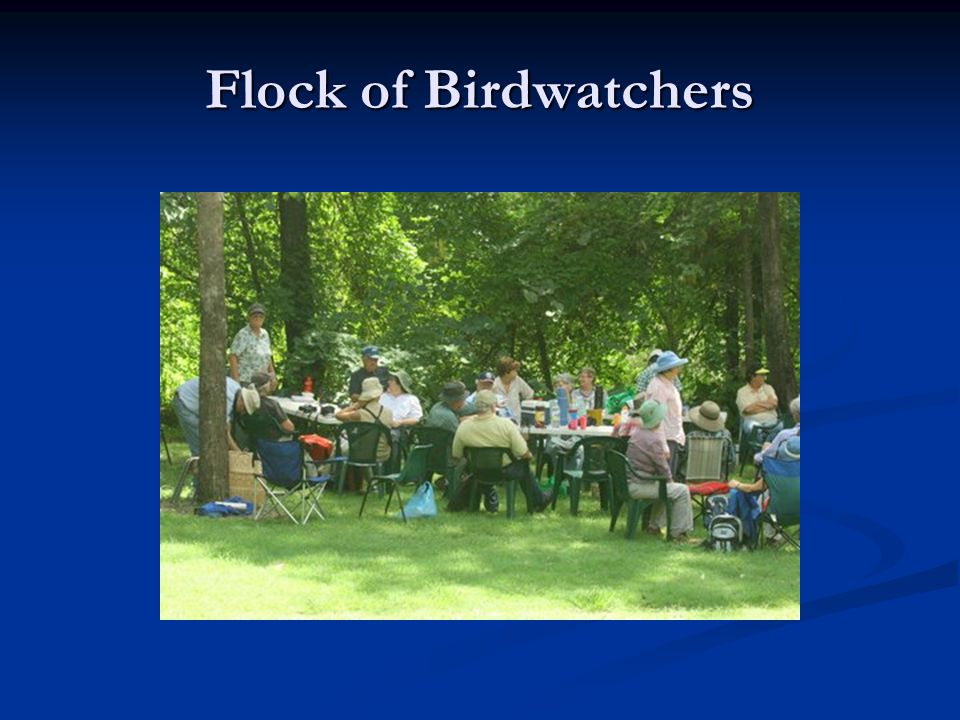The image is framed by a medium blue border, which gradually darkens towards the top. Centered at the top of the border, bold white text reads "FLOCK of BIRDWATCHERS," with the 'F' and 'B' notably capitalized. Within the frame is a color photograph depicting a lively scene on a well-trimmed grassy lawn, surrounded by trees. Around 15 to 20 people are gathered, seated on portable chairs and around fold-out tables adorned with binoculars, food, and drinks, suggestive of a picnic setup. The participants, men and women of various ages, are equipped with sun hats, sun visors, and ball caps, indicating they are prepared for an outdoor birdwatching activity. Some individuals are standing, while others have their backs turned to the camera, adding to the candid atmosphere of the gathering.